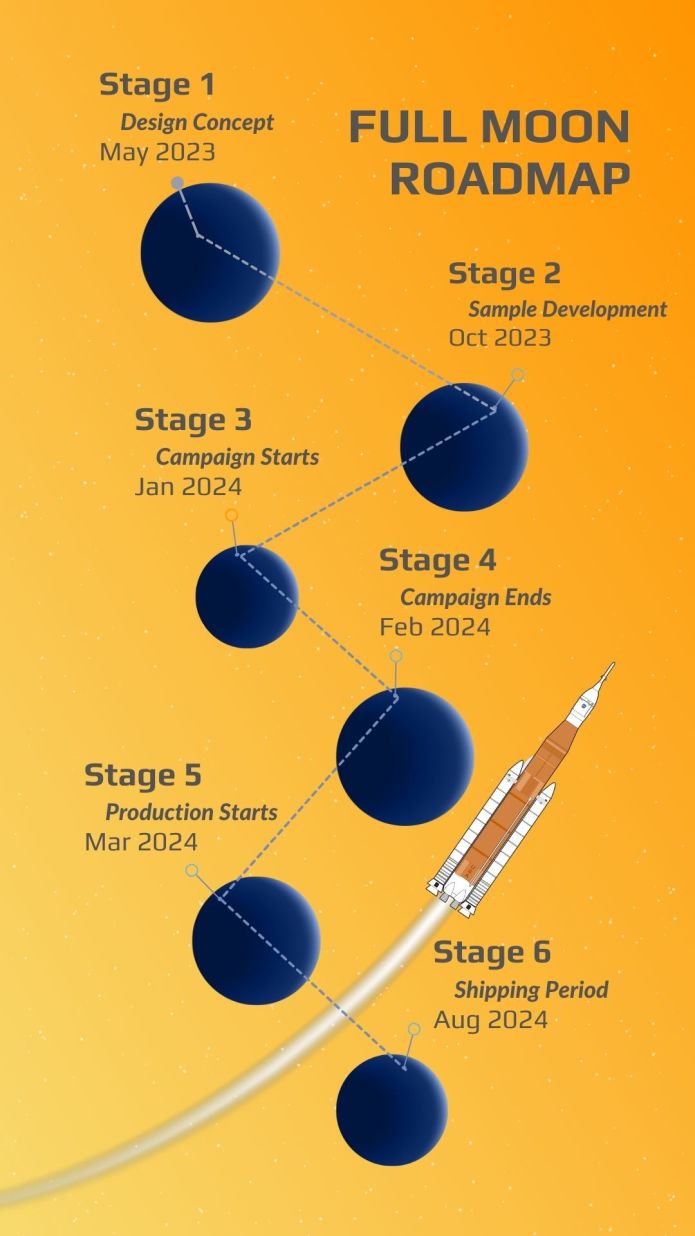The image is a rectangular chart titled "Full Moon Roadmap" in bold gray text at the upper right-hand corner, with dimensions approximately six inches high and three inches wide. The background transitions from dark orange at the top right to a pale yellow toward the bottom left. It features a zigzag pattern of six blue circular stages connected by a dotted blue line. Each circle has a specific stage and date labeled in gray text: 

- **Stage 1**: Design Concept (May 2023)
- **Stage 2**: Sample Development (October 2023)
- **Stage 3**: Campaign Starts (January 2024)
- **Stage 4**: Campaign Ends (February 2024)
- **Stage 5**: Production Starts (March 2024)
- **Stage 6**: Shipping Period (August 2024)

A rocket with two boosters is depicted coming from the bottom left and ascending between the moons, emphasizing a progress trajectory. The visual elements, including the consistent blue circular stages and dotted line, guide the viewer's eye through the timeline in a dynamic zigzag formation. Each moon’s size is mostly uniform, except for subtle variations in the third and final stages.